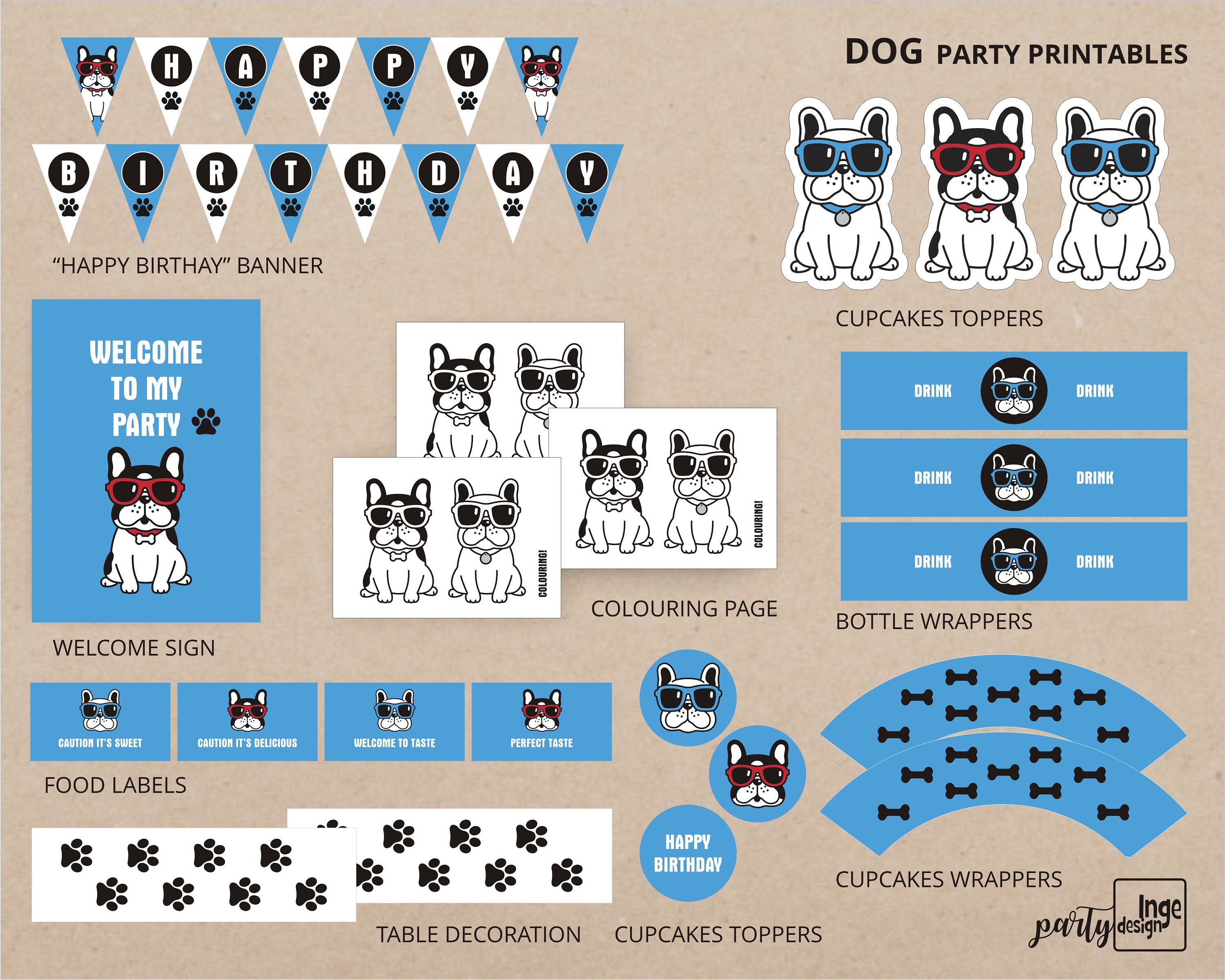This landscape poster, set against a beige-brown background, showcases a variety of party products centered around a dog theme. Dominating the upper portion is a bold title in black text, "Dog Party Printables." Just beneath, a banner with alternating blue and white triangular flags spells out "HAPPY BIRTHDAY," each letter encased in a black circle with white lettering, accompanied by black paw prints. The eye-catching dog motif prominently features a pug-like dog sporting blue or red sunglasses.

Beneath the banner, multiple cutouts detail various party items: 
- A blue card stating "Welcome to my party" with a dog and a paw print.
- Rectangular and circular table decorations and bottle wrappers, many depicting dog faces or paw prints.
- Cupcake toppers and wrappers adorned with dog bones, adding charm to party treats.

The majority of images and text on the poster follow a blue and white color scheme, enhancing the cohesive look. Additionally, there's a coloring page for younger kids, all on a neat layout meant for easy cutouts. This poster highlights an array of party essentials, perfect for a children's dog-themed celebration.